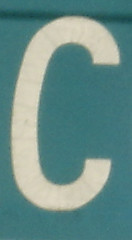The image features a vertically aligned, narrow rectangular area on a white background. The main portion is a light greenish-blue color. A large, somewhat worn white block letter "C" dominates the center of this background, spanning almost the entire height of the rectangle. Directly above the letter "C," near the top of the image, runs a dark green horizontal stripe. This stripe appears to be part of the surrounding surface, which resembles a medium blue-painted wall or sign. The white letter "C" itself has flat, simple ends and is angled very slightly to the right, potentially due to the photograph's perspective. Overall, the image conveys the impression of an exterior shot of a weathered sign or painted surface.